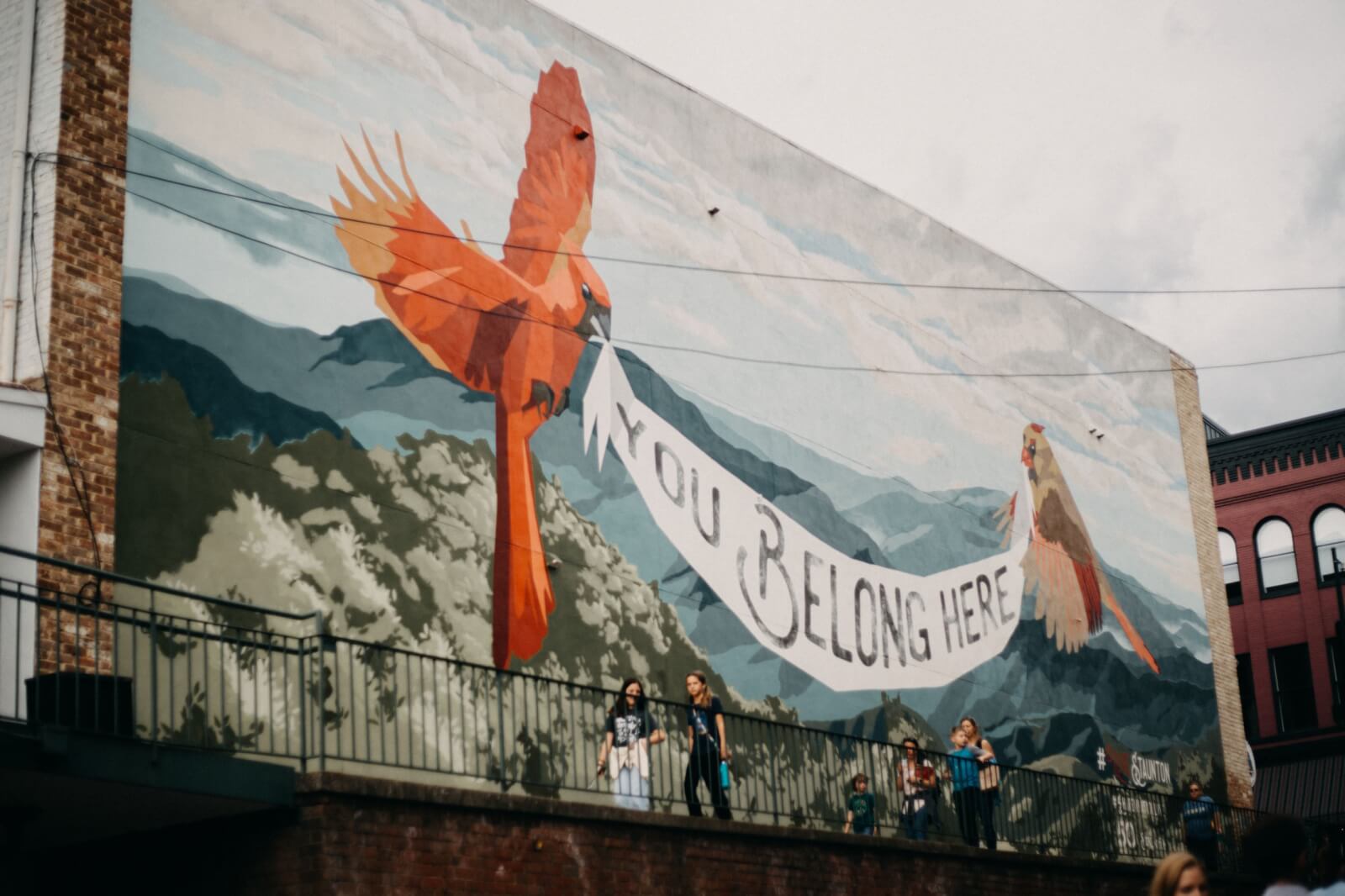The image showcases a vibrant mural painted on a brick wall in a cityscape. This mural, also bordered by visible dark red bricks on the left side and at the bottom, artistically depicts two birds soaring in a sky filled with light blue and patches of white clouds, painted above a mountainous landscape that possibly features snowy peaks. On the left, the bird, likely a male cardinal, is adorned in striking hues of red and orange, while the bird on the right, possibly a female cardinal, features a more subdued palette of tan, off-white, with touches of peach and red. Both birds hold a white banner in their beaks that lovingly declares, "You belong here." In front of the mural, a black handrail spans across its bottom edge, creating a subtle boundary. Between the handrail and the mural, several people are casually walking, with two young ladies—one notably holding a turquoise water bottle—appearing prominently. The day itself seems overcast, completing the scene with a soft, diffused light that complements the mural's engaging warmth and invitation.